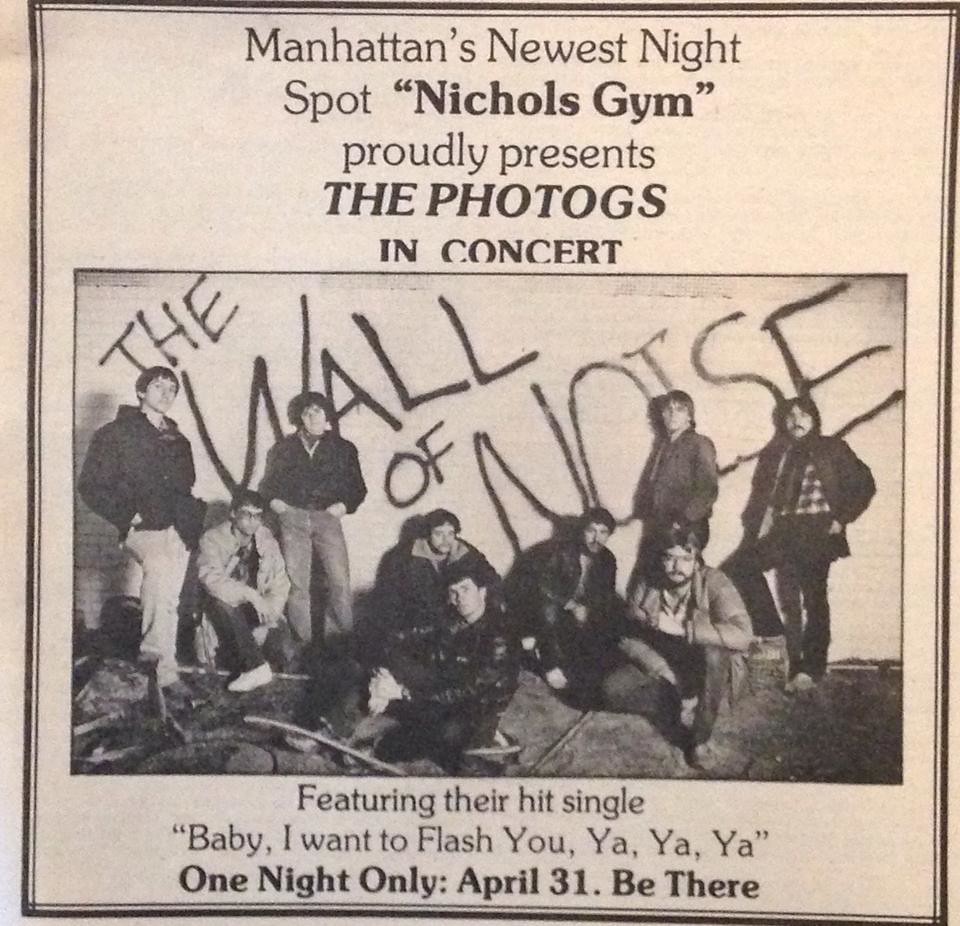This image appears to be a vintage newspaper advertisement for a concert. The ad is framed with a black border and has an overall aged, dingy appearance, with the background having a faded pink tint, giving it a grainy, old look. At the top, the text reads, "Manhattan's newest night spot, Nichols Gym, proudly presents The Photogs in concert." 

The central feature of the ad is a large black-and-white photo depicting nine band members, some standing and some sitting among rubble, against a brick wall. The wall is adorned with graffiti-style writing that says "The Wall of Noise." Below the photo, additional text promotes the band's hit single, "Baby, I Want to Flash You, Yeah Yeah Yeah," and announces, "One night only, April 31. Be there." The ad, with its double-bordered frame and detailed descriptors, exudes a nostalgic and rustic charm.